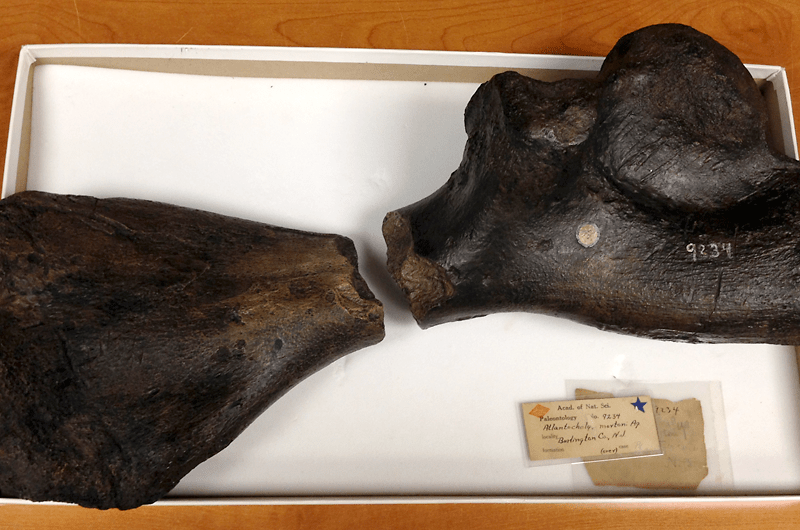This photograph showcases an artifact, likely an ancient fossil or bone, separated into two distinct pieces and placed in an upside-down white shoebox lid, serving as a tray. The dark brown, triangular-shaped fragments are meticulously positioned on a white fabric lining the bottom of the box. The bone piece on the right is clearly marked with the number "9234" or "9334" in white digits. Accompanying the artifact, at the bottom right corner of the tray, is a laminated label bearing cursive writing that includes the location "Burlington, New Jersey." This label features a blue star in the top right corner and an orange or gold triangle in the top left corner. The entire setup rests on an orangish-brown table, suggesting a controlled environment, possibly for inventory or cataloging purposes in a museum or archaeological study.